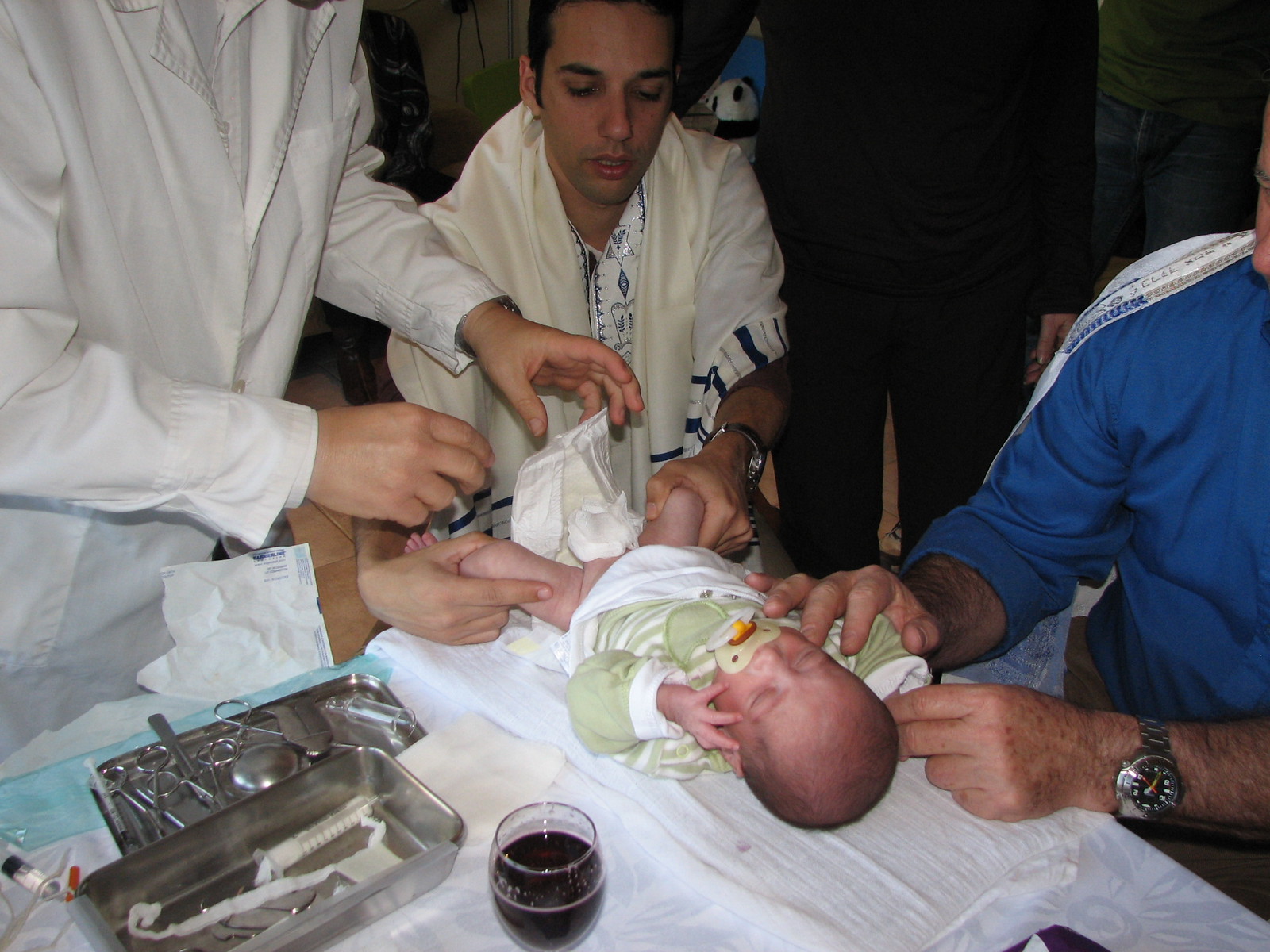The image depicts a Jewish family performing a bris ceremony, a traditional circumcision. The central focus is a newborn baby lying on a white, clean medical sheet, with a green pacifier in his mouth and dressed in a green shirt. The baby's diaper has been removed and there's white gauze covering the genital area. To the bottom left of the frame, there are sterile trays filled with medical tools, including scissors. 

In the lower part of the image, there's a dark red glass of wine. Surrounding the baby are several figures, including a gentleman in white with a white scarf looking down at the baby, who might be officiating the ritual. Another person in a white medical lab coat is tending to the baby, possibly bandaging or putting the diaper back on. Additionally, there's a man in a blue shirt with a silver watch holding the baby's hand while a figure mostly hidden in black stands in the background. The overall setting appears to be a table or kitchen table, typical for such intimate family rituals.